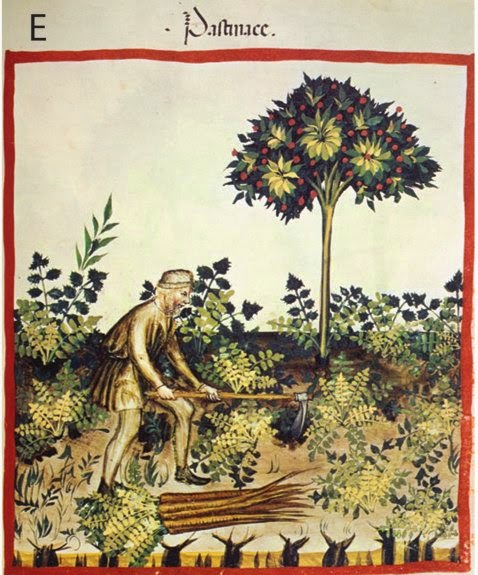The image depicts a vintage-style painting bordered with red, featuring the letter "E" in the top-left corner and an inscription in an unreadable, non-English script above it. At its center, a figure, likely a man dressed in a tunic and tights with a hat, is engaged in cultivation, using a hoe to dig up carrots in a tan-colored garden. The ground is scattered with horizontally lying wood and newly harvested carrots. To the right, higher up, stands a narrow-trunked tree with green leaves and red and yellow elements that resemble fruit, adding an abstract touch to the scene. The background is predominantly tan, emphasizing the earthy tones and activities within the garden.